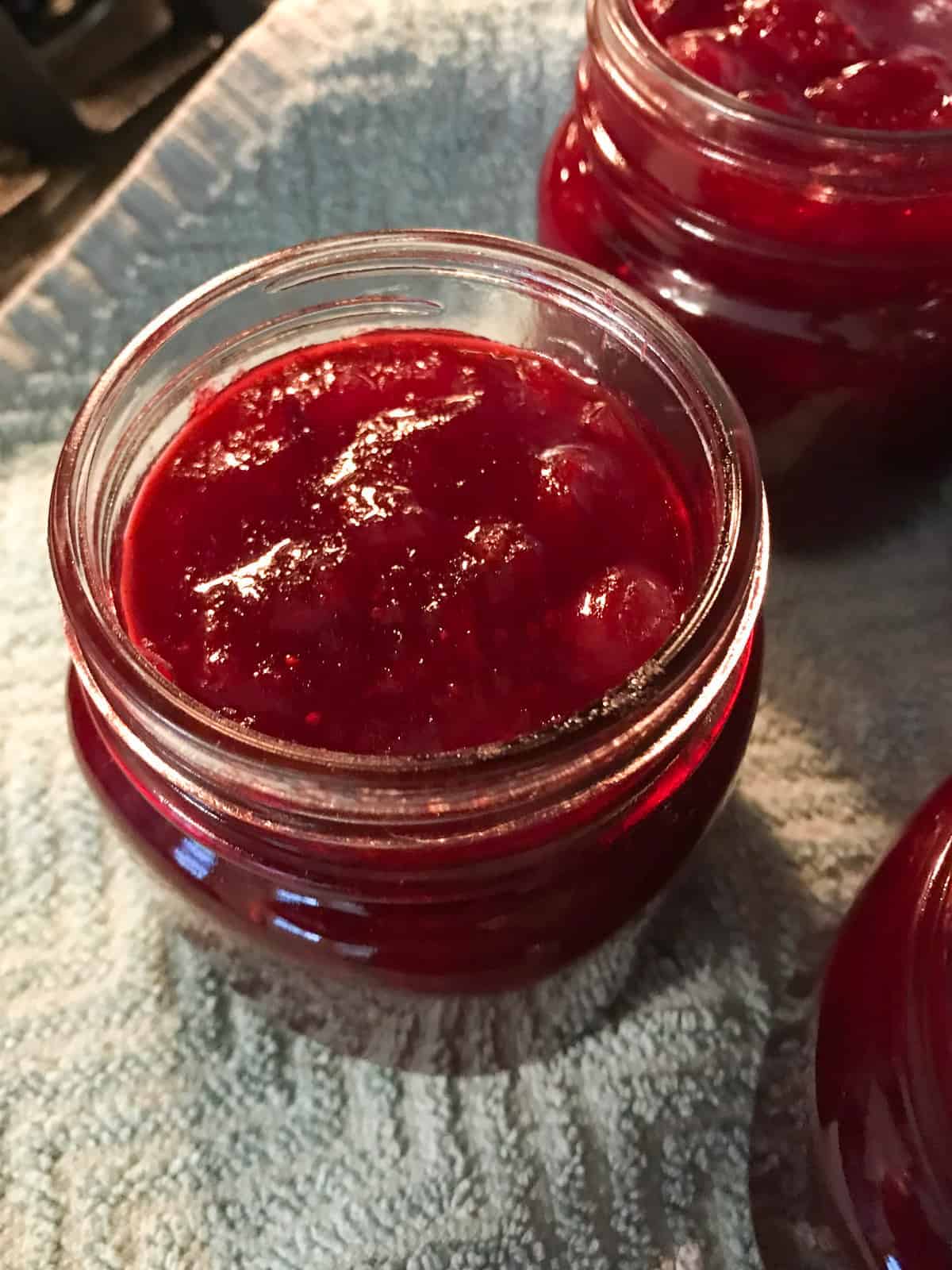The image shows a close-up view of three glass jars containing a red fruit preserve, likely strawberry or cherry jam. The central jar, which is fully visible and slightly to the left of the frame, has an open top, displaying its thick, jelly-like contents with identifiable fruit pieces and possible seeds. The other two jars are partially visible—one situated towards the upper right and another towards the lower right. These jars lack labels and have the threading for lids, though none are present. The jars rest on a textured, light blue tiled surface that appears to be a kitchen towel, and a small segment of an indistinguishable dark surface is visible in the upper left corner of the image. The light source seems to come from behind, illuminating the tiles and enhancing the translucency of the jam.